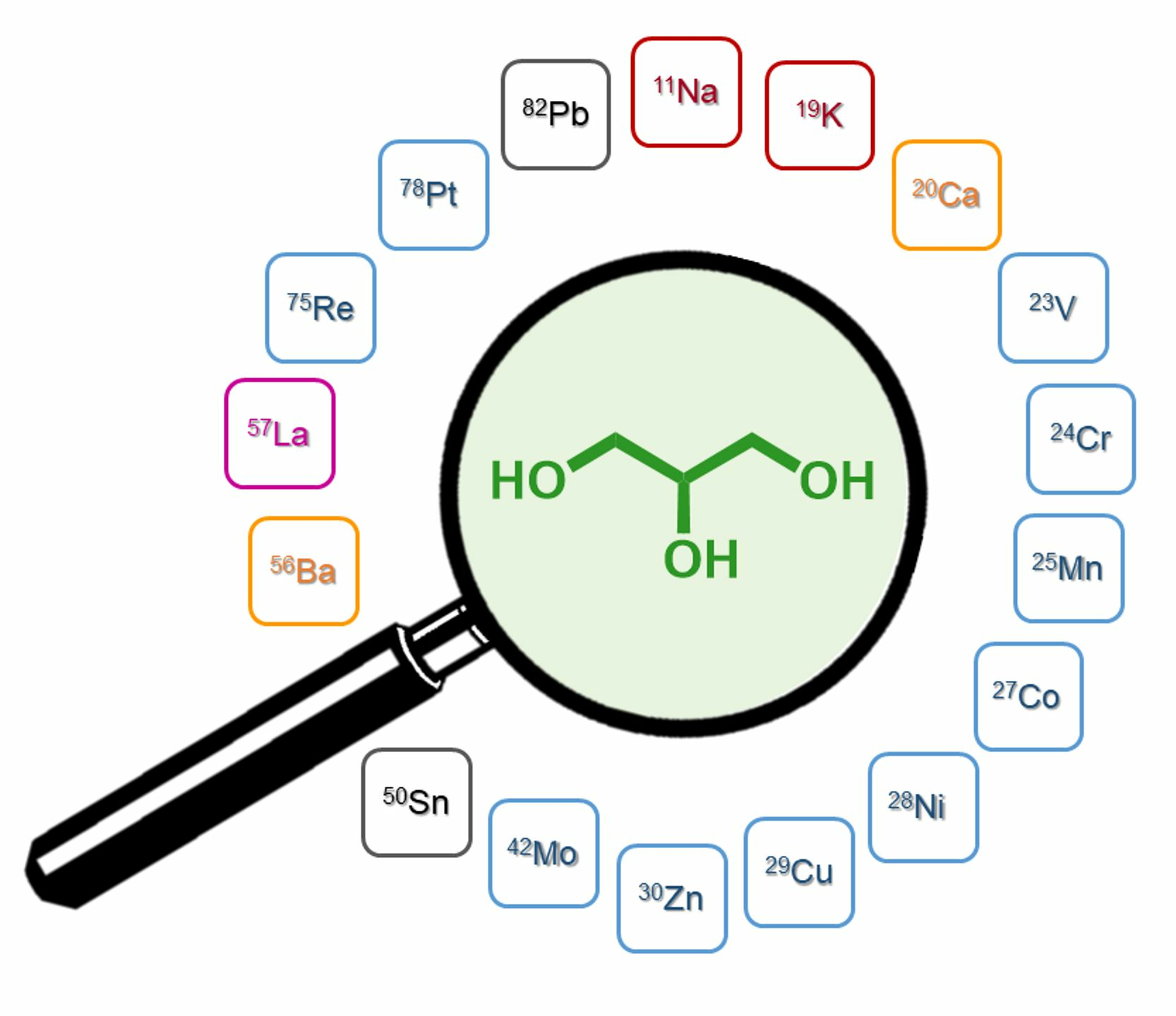The image is a detailed graphic visual art piece with a white background featuring a black magnifying glass prominently centered. The magnifying glass has a dark handle that extends from the bottom left, displaying highlights, and a black border around its circular lens. Inside the lens, the background is a light green, framing a molecule diagram with three branches. Each branch is marked at the end with the group "OH," connected by a green line. The molecule also features the word "HO" on the left, "OH" in the middle, and another "OH" on the right.

Encircling the magnifying glass are various squares, each representing a different chemical element from the periodic table, complete with their symbols and atomic numbers. These squares are color-coded in shades of orange, pink, black, blue, and red, and each has curved corners. The displayed elements include notable symbols such as "11NA" in the top middle and "19K" to its right, among others like zinc and copper. The vivid and educational nature of the image, combined with its animated style, suggests that it could be an illustration from a chemistry textbook cover.